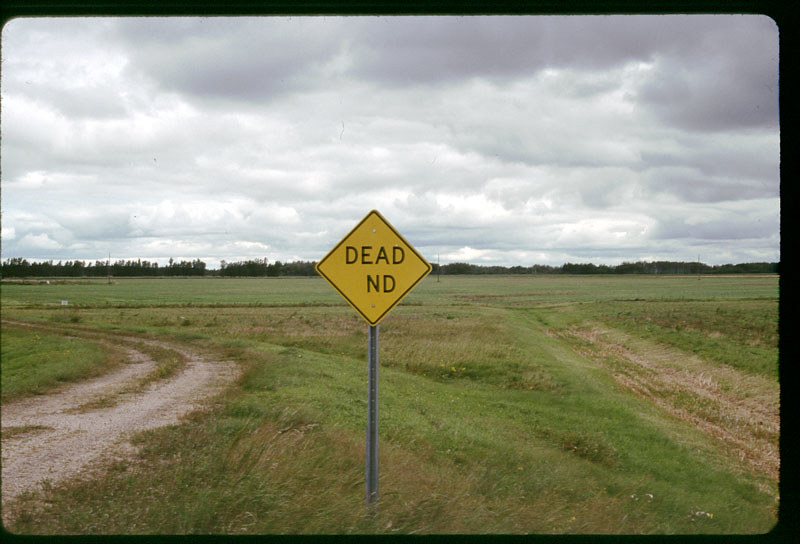A weathered, yellow diamond-shaped sign stands forlornly at the confluence of two dirt roads, seemingly abandoned between the splits of the paths. Its intended warning of "Dead End" is marred by the missing "E," leaving only "Dead N D" in bold black letters. Mounted on a rusted silver metal post, the sign emerges from a clump of overgrown grass. The dusty dirt roads meander away from the lower corners of the image—one curving from the bottom left towards the center-left, the other extending straight from the lower right to the mid-right—forming a subtle Y-shape. The scene is set against a field stretching into the distance, bordered by a line of dense trees that stand uniform from left to right. Above the trees, heavy gray clouds loom, casting a melancholic shadow over the entire landscape. The image encapsulates a quiet, almost eerie isolation, frozen in time.